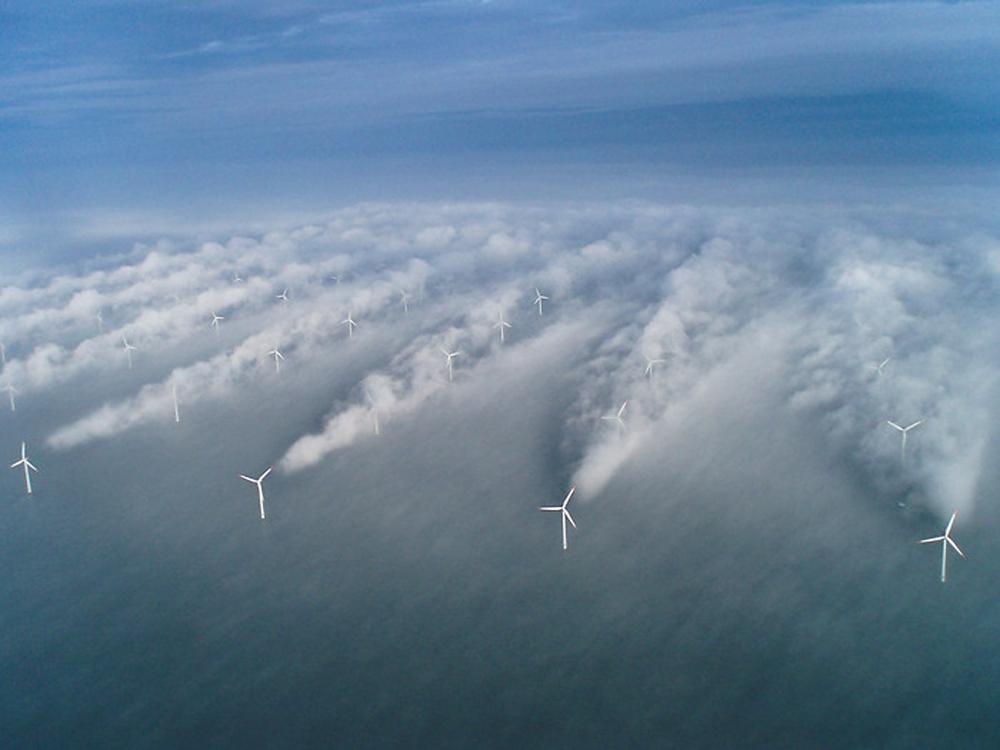This photograph captures an intriguing aerial view of a vast wind farm, displaying dozens of evenly spaced white windmills. Taken from above, the perspective brings a unique and somewhat surreal aspect to the scene. The windmills appear to be emerging from or nestled within a dense, smoky layer of clouds, creating an illusion that blends earth and sky. The scene is further punctuated by the motion-blurred, rippling trails of clouds that give a sense of dynamic movement across the windmills. Above this ethereal landscape, the sky remains mostly blue with a few thin wisps of clouds, adding to the dreamlike quality of the image. The overall effect raises questions about the photograph’s authenticity, suggesting the possibility of artistic manipulation to enhance the otherworldly atmosphere.